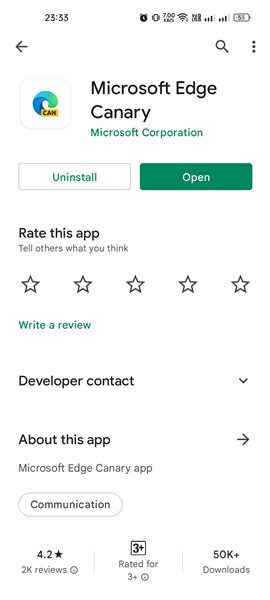Screenshot of Microsoft Edge Canary App's Google Play Store Page

This screenshot, captured from the Google Play Store, features an all-white background with a detailed display of the Microsoft Edge Canary app page on a smartphone.

### Top Bar and Status Indicators
- **Time Display:** The top left corner shows the time, "23:33".
- **Battery Icon:** Located in the top right corner, the battery icon displays 55% charge.
- **Connectivity Icons:** Two Wi-Fi or Internet connectivity icons are present, with three of the four bars filled.
- **Additional Icons:** To the right, an unreadable lettering is visible. Indicators for Wi-Fi, an alarm set for 7:00, phone on vibrate mode, and an alarm icon follow in succession.

### App Information Section
- **Navigation Arrow:** Positioned on the left side, there's a black back arrow.
- **Search and Menu Icons:** Underneath the battery icon, there are a search magnifying glass and a vertical three-dot menu icon.
- **Microsoft Edge Canary Details:**
  - A small white square featuring the Microsoft Edge icon is below the back arrow.
  - To the right, "Microsoft Edge" is written in bold black lettering.
  - Below, "Canary" is written in black.
  - Further down, "Microsoft Corporation" in a teal green font.
  
### Interaction Buttons
- **Uninstall and Open:** 
  - On the left, a green button labeled "Uninstall".
  - On the right, a green button labeled "Open" with white text.
  
### User Feedback Section
- **Rate and Review:**
  - An inch below the "Uninstall" button, "Rate this app" appears in black text.
  - In smaller black text, the prompt "Tell others what you think."
  - Below, five outline circles, representing the rating scale.
  - To the left, in green text, "Write a review".
  
### Additional Information
- **Developer Contact and About:** 
  - "Developer contact" is written in black beneath a small space.
  - A bit further down, "About this app" appears in smaller black text, with the Microsoft Edge Canary description.
- **Category and Reviews:**
  - Below, a tab indicating the category, "Communication," in black text.
  - At the bottom, sections display user reviews, the number of reviews, the app's age rating, and the download count.

This comprehensive view provides users with essential app information, enabling easy navigation and interaction with the Microsoft Edge Canary app on the Google Play Store.